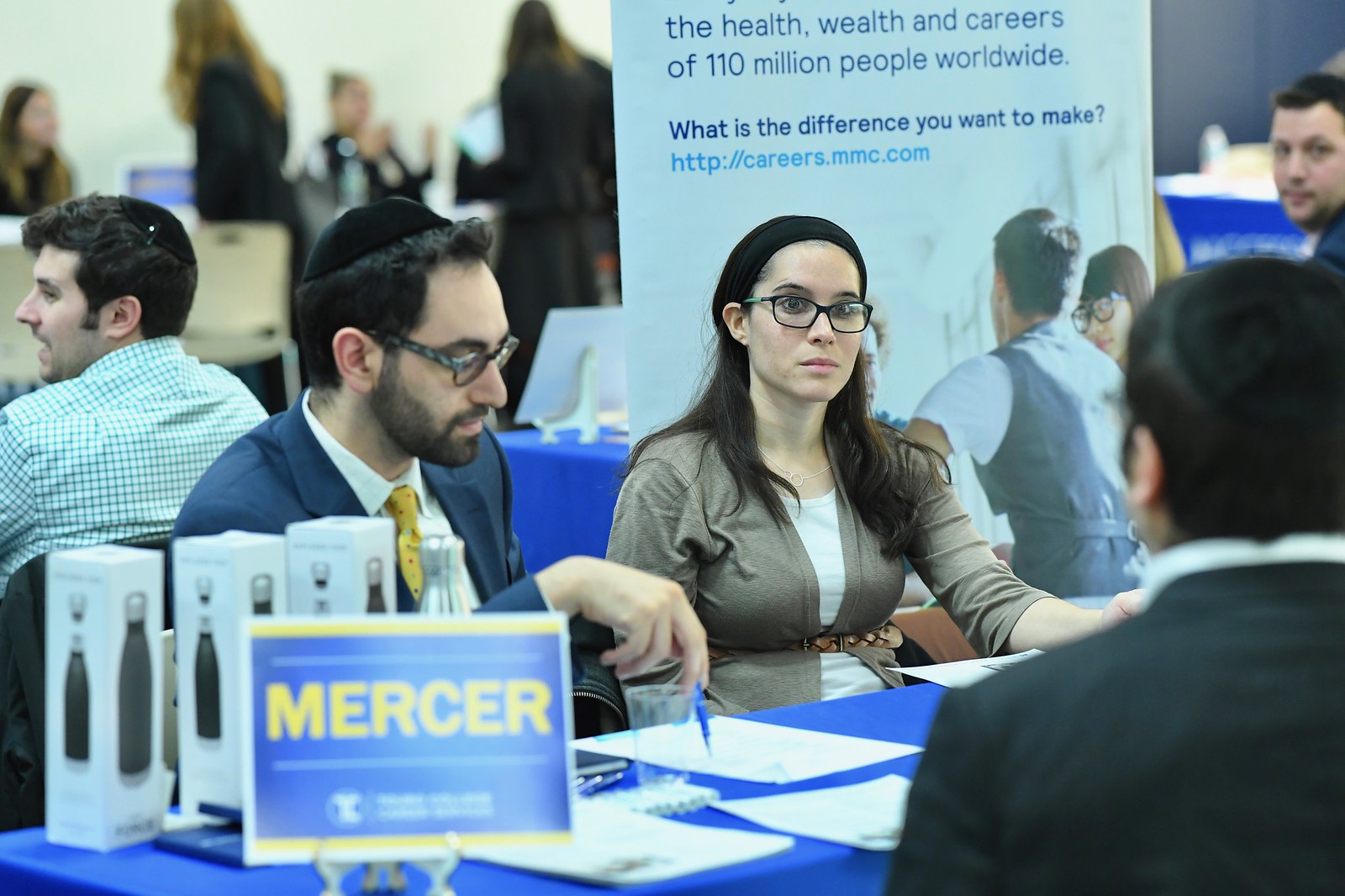This color photograph captures a scene inside a conference hall, possibly in New York City, during a career fair or a professional event. The central focus is a bearded man in his 30s or 40s, wearing a black yarmulke, a suit, a white shirt, and a yellow tie. He sits at a table covered with a bright blue tablecloth, holding a pen poised over a piece of white paper. To his right, a young woman with shoulder-length black hair, glasses, and wearing a long-sleeved jacket over a white shirt and belt, engages in conversation with another man across the table. The table prominently displays a sign with the word "Mercer" in yellow letters on a blue background, possibly indicating a connection to Mercer University or the Mercer consulting firm. Behind them, a banner reads, "The health, wealth, and careers of 110 million people worldwide. What is the difference you want to make?" followed by a URL: http://careers.mmc.com. In the background, some attendees are blurred, while a young man in a checked shirt, seen in profile, is in focus, conversing with someone. Also visible are boxes likely containing giveaway water bottles. This photographic composition effectively captures the collaborative and professional atmosphere of the event.